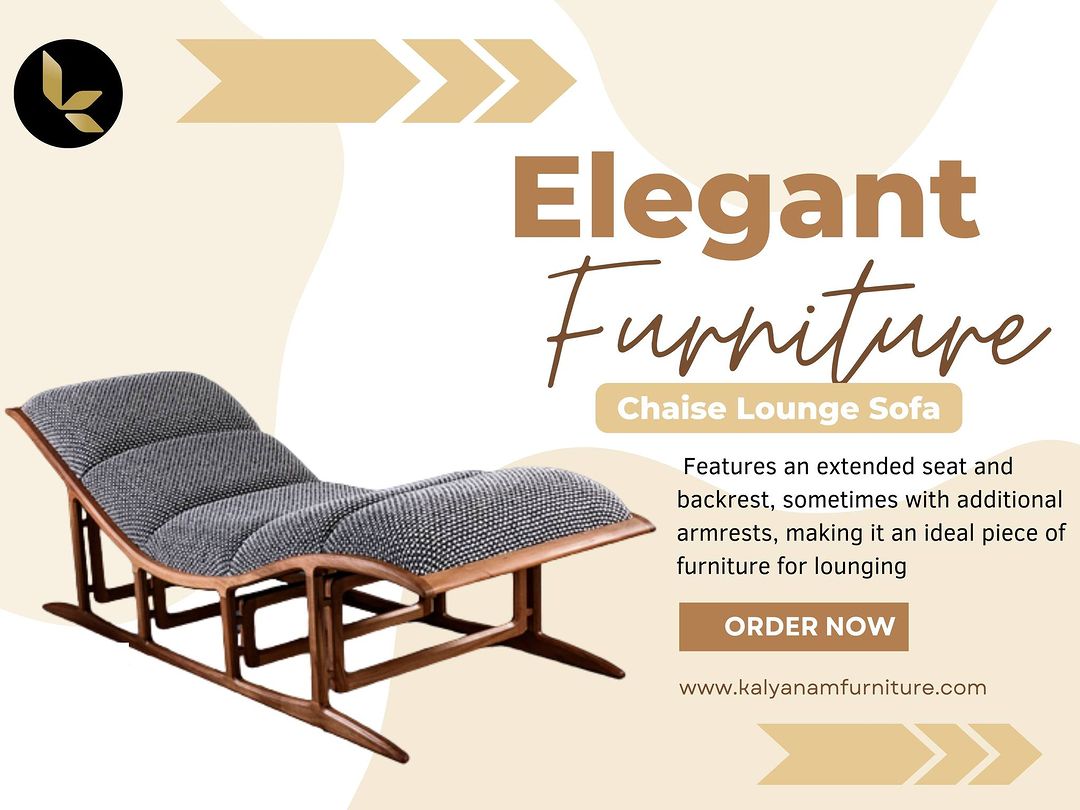The advertisement, designed with a salmon and white background featuring salmon-colored lines, showcases a blend of elegance and functionality. At the top left, a black circle with a golden logo subtly draws the viewer's attention. Dominating the upper right corner, "Elegant Furniture" is prominently displayed, with "Elegant" in bold orange text and "Furniture" in cursive brown text.

The centerpiece of the ad is a detailed illustration of the featured item, the Chaise Lounge Sofa. This piece of furniture, perfect for lounging, combines comfort and style with its unique design. The sofa features five dark blue rectangular cushions adorned with white dots arranged in a grid pattern. These cushions rest on a curved rectangular base, which elegantly dips at the ends. Supporting this structure are sleek dark wood legs interconnected by a rectangular frame with a central space, enhancing its stability and aesthetic appeal.

Highlighting its offer, the ad presents the name of the furniture piece and a call to action in clear text: "Order Now." The chaise lounge sofa is described as the ideal furniture for extended seating and backrest comfort, sometimes complemented with additional armrests. The advertisement includes the website's address, www.kalyanamfurnitures.com, in black text at the bottom right, inviting potential buyers to explore and purchase this elegant piece.